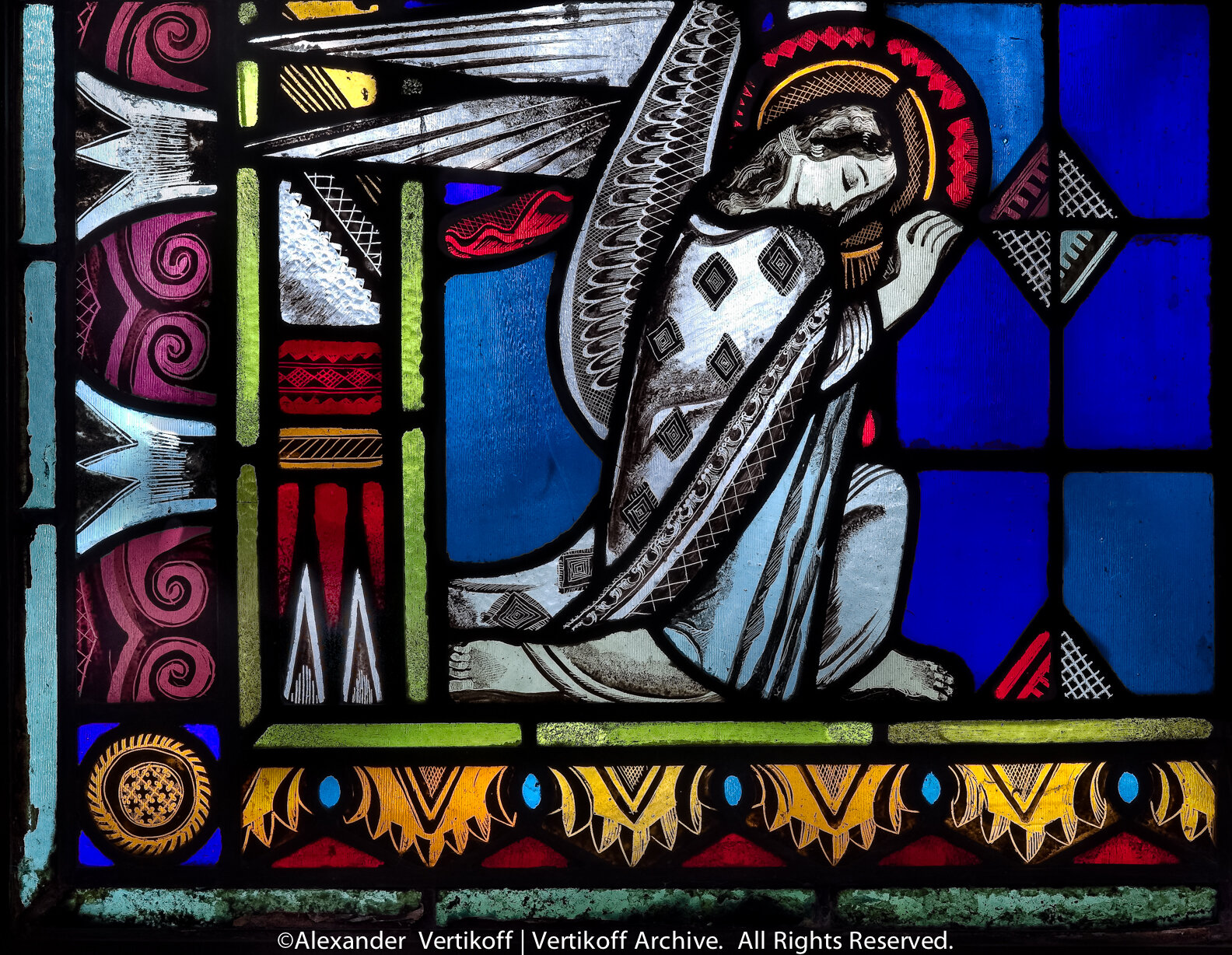This image captures a highly detailed section from the lower left-hand portion of a stained glass window, potentially seen in an old-fashioned church. Central to the image is a depiction of a kneeling angel or female religious icon with dark hair, facing right and bent forward in prayer. The figure's head is adorned with a vibrant halo encircled by red symbols, yellow outlines, and a black etching, adding depth to the celestial depiction. A tall set of wings extends upward from the figure’s back, blending into the deep cobalt blue background segmented by black framing typical of traditional stained glass work. 

The borders of this section are richly decorated. The left edge features elaborate red, white, and green patterns resembling crowns, interspersed with turquoise bars that appear age-worn or artistically distressed. Further intricacies appear in the lower left corner, where a distinguishing emblem with a cobalt blue background and a yellow fleur-de-lis pattern within a black circle stands out. Adjacent to this, the lower frame showcases yellow designs draped over a red background, contributing to the ornate framing.

At the bottom of the image, a black border contains a clear copyright notice: "Copyright Alexander Vertikoff, Vertikoff Archive, All Rights Reserved." The striking colors and meticulous detailing suggest that this could either be a photograph or an artistic rendition of a stained glass window, though the exact nature remains ambiguous.